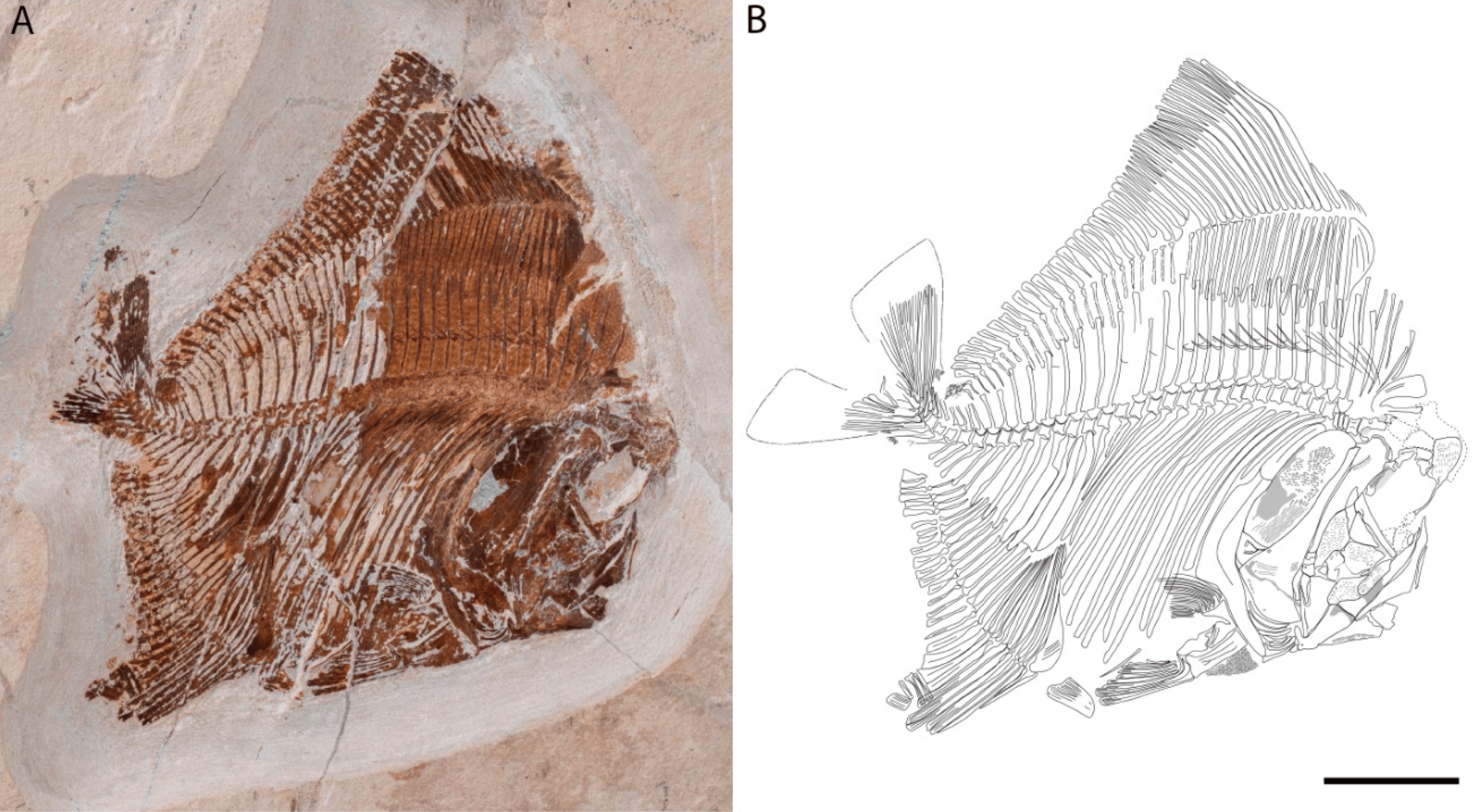The image consists of two side-by-side panels labeled with letters in the top left corners. The left panel, labeled with a black "A," features a photograph of a fossilized fish encased in a pale stone or sandstone, meticulously smoothed around the fossil to fully expose its details. The fossil, a brown imprint within the stone, reveals the vertebrae, fins, and eye of the fish. The right panel, labeled with a black "B," presents a detailed black-and-white pencil drawing of the same fossil. This illustration focuses solely on the bones and structure of the fish, omitting any background representation of the stone. Both images are likely sourced from an archaeological or paleontological context, with the photograph providing a realistic view and the drawing offering a more precise anatomical depiction.